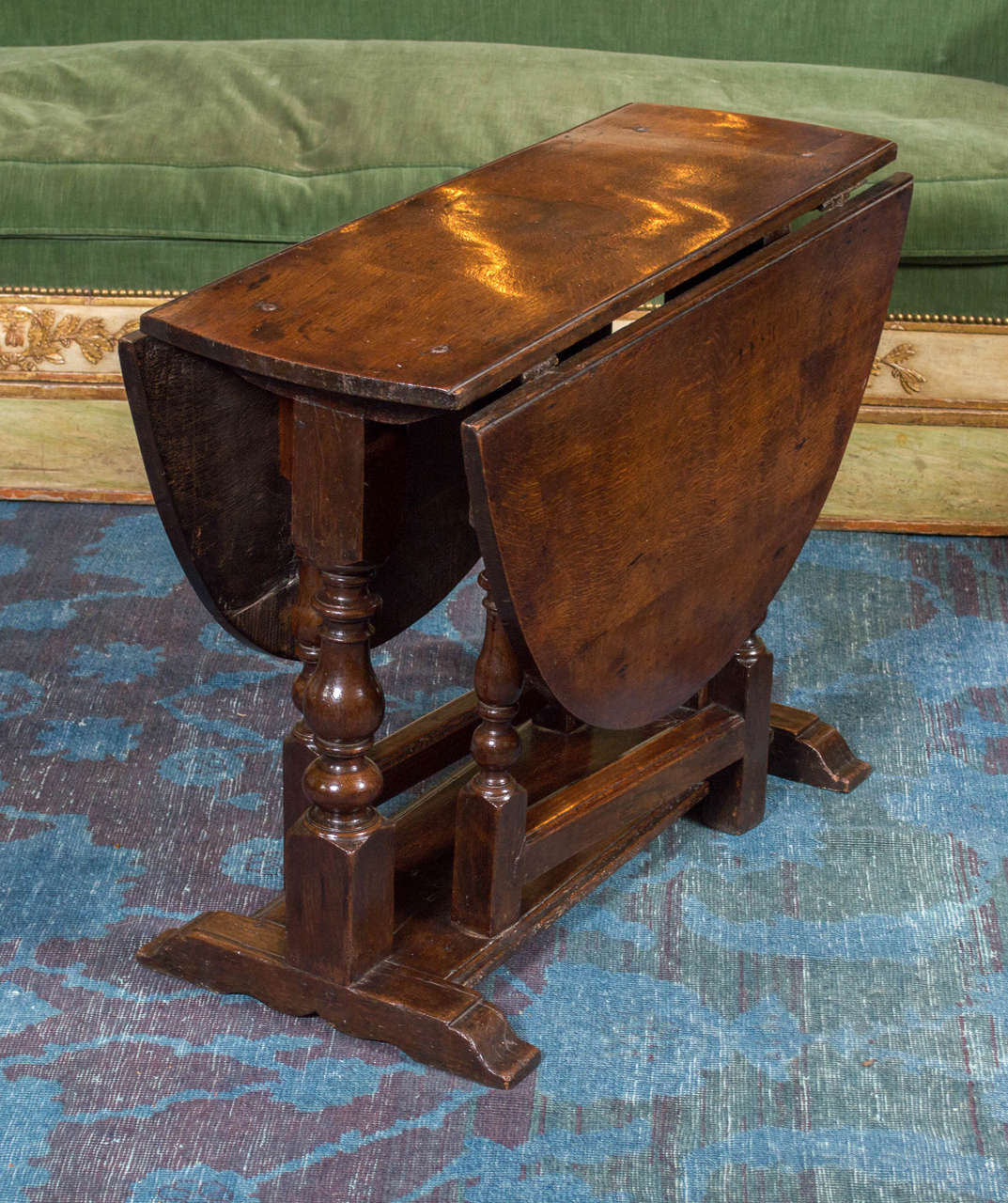The photograph depicts a detailed indoor living room scene centered around a vintage, foldable wooden table. The table is primarily brown with a shiny finish, featuring two rounded flaps on either side that have been folded down, revealing only the central section. Its legs are intricately designed, with squared top and bottom parts and decorative circular embellishments in the middle. The table stands on a distinctive carpet that is predominantly blue, interspersed with gray and dark red splotches. In the background, an older green couch with a stained cushion is visible. The couch has a wooden frame adorned with a leafy design, adding to the retro ambiance of the room. There are no people present in the image, allowing for a focused view of the furniture and decor.